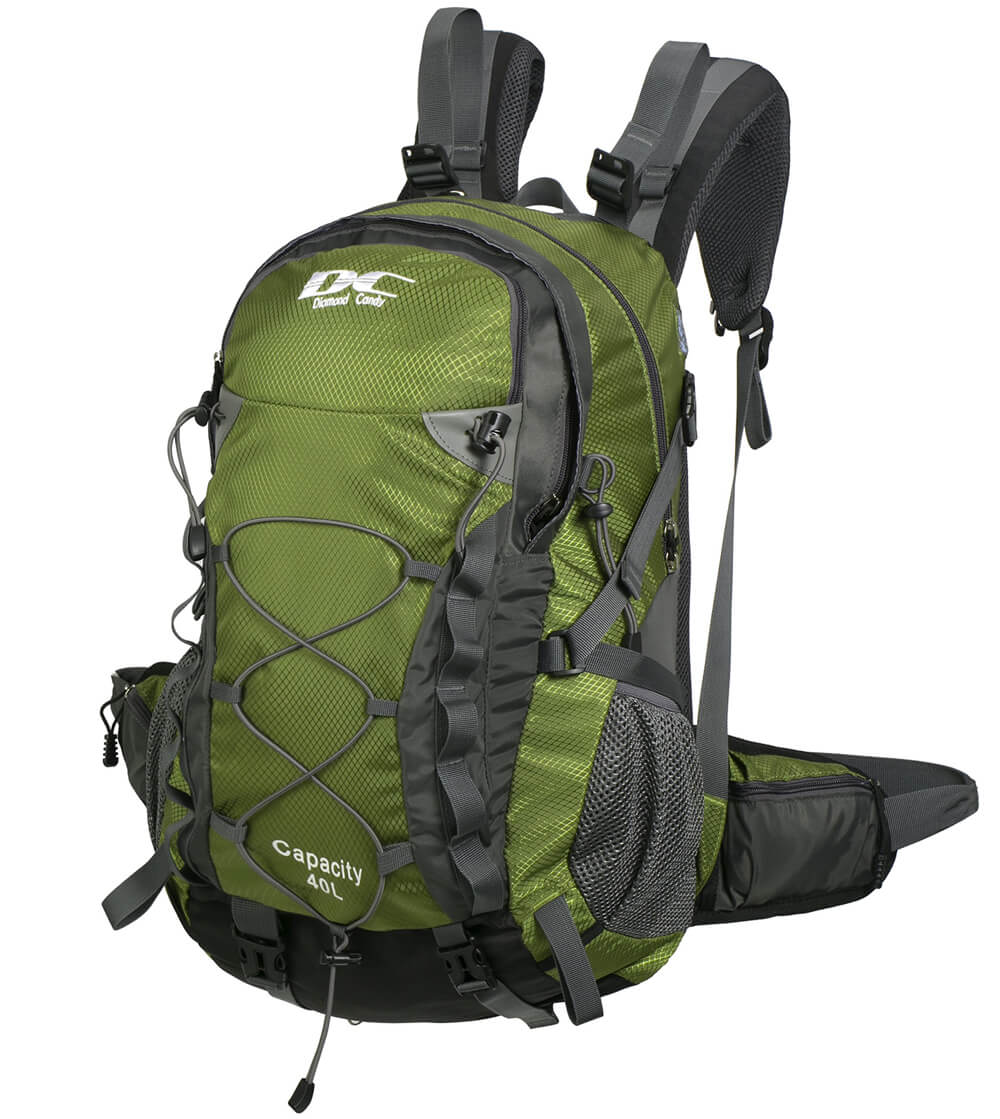This is a detailed color photograph of a dark green hiking-style backpack, featuring black and gray accents. The backpack, which appears to be a stock image possibly for online retail like Amazon.com, prominently displays the brand name "Diamond Candy" with the initials "DC" at the top. The middle section of the backpack states its capacity as "40 Liters" or "40L" in white lettering. The backpack is equipped with multiple compartments, including various zippers, pockets, and drawstrings. It has a mesh side pocket on the right and a gray cord running down the middle. The straps, designed for comfort, are black and padded, extending around the shoulders and waist. The image solely focuses on the backpack, with no people, animals, or buildings visible in the background.